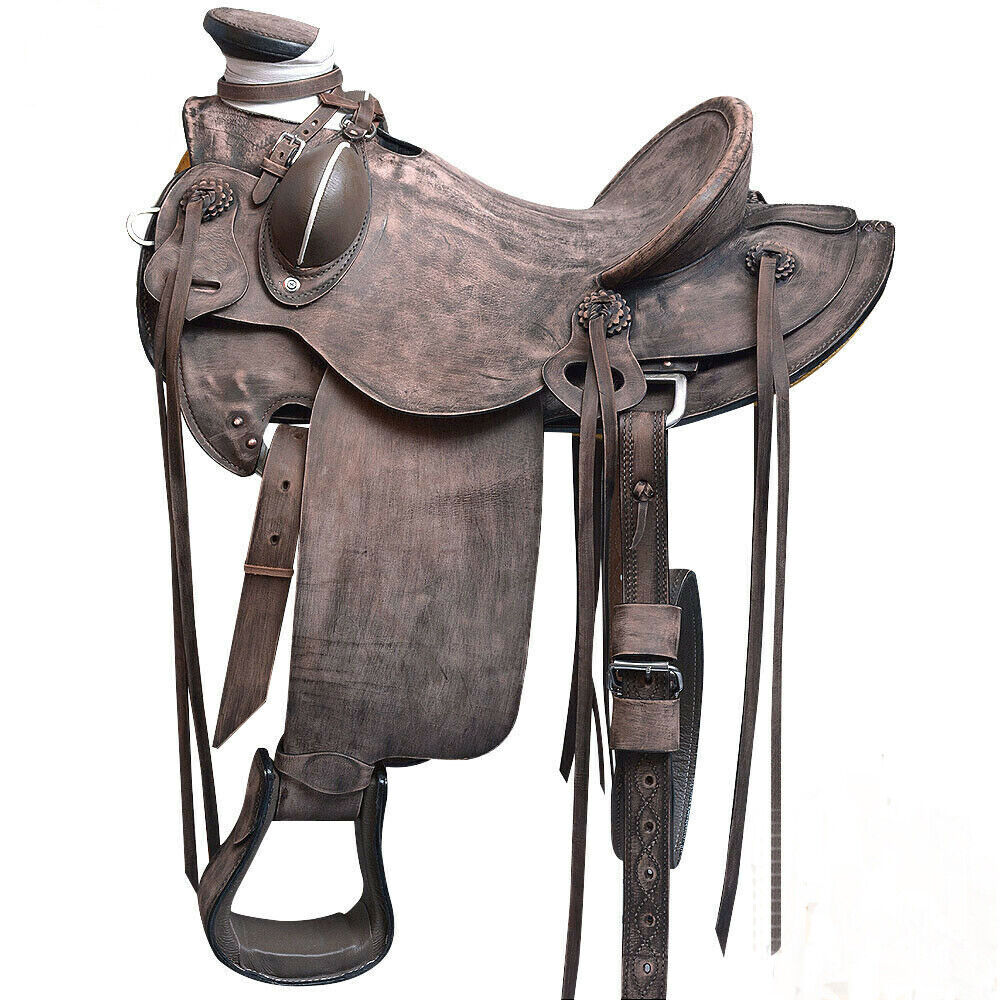The image depicts a well-worn, vintage horse saddle made primarily of thick, stiff brown leather with mottled black areas and subtle hints of gray and pink. The saddle, positioned against a pure white background and viewed from the left side, shows signs of extensive use and weathering. At the front, there is a prominent black handle, or horn, wrapped in white cloth and secured with leather straps. Surrounding the horn are various belts, buckles, and leather tassels. The seat features a high arch at the back to support the rider, preventing them from falling off. Additionally, the back of the saddle has thin leather straps hanging from a brass rivet, possibly intended for use with the horse. The saddle is adorned with various leather ties and streamers, enhancing its intricate and rugged appearance.